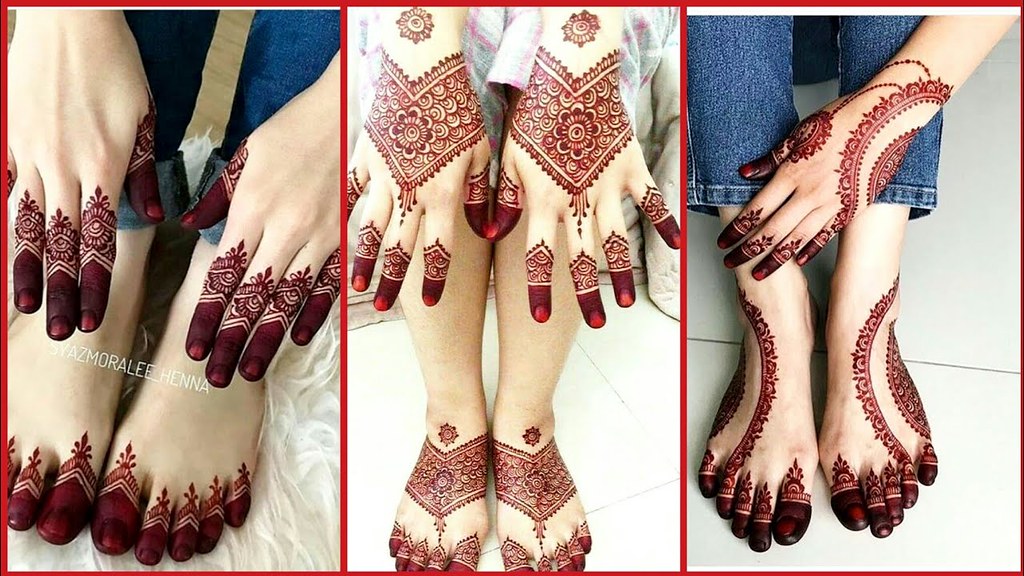The image is a triptych of three photographs, each framed with a red border, showcasing intricate henna designs on the hands and feet of what appear to be three Caucasian females. In the first photograph, the woman's feet are adorned with extensive henna designs, completely covering her toes and extending up her feet. The henna on her hands similarly covers her fingertips and extends down her fingers to her palms. A watermark indicates the henna artist as Yaz Morali. The second photo features another woman with henna designs reaching up to her ankles and wrists. Her feet have elaborate patterns culminating in floral designs at the ankles, while her hands showcase intricate henna extending from fingertips to wrists. The third image displays a woman with a distinct curvilinear henna design on the upper portions of her feet, extending up to her ankles, with coverage on the sides of her feet as well. Her lone visible hand sports a similar pattern, characterized by branches that form a complex floral motif ending near the thumb. She is dressed in jeans, in contrast to the second individual who appears to be wearing shorts. The dominant color of the henna across all images is a dark red, emphasizing the elaborate and detailed artistry of each design.